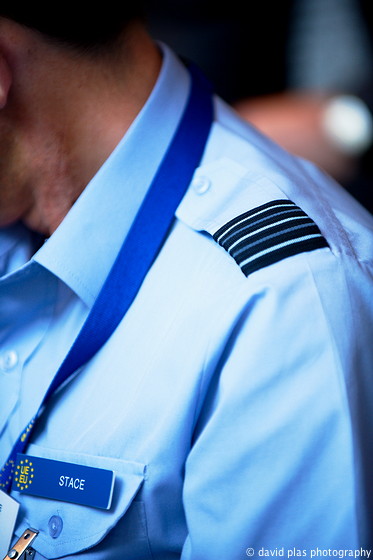This close-up photograph captures a man, likely an airline pilot, dressed in a light blue shirt with a neatly buttoned white button on a light blue collar. He is turned slightly to the left, offering a partial view of the back of his head, where his black hair is visible, and the front of his shirt on the left edge of the image. A dark blue lanyard hangs around his neck, supporting a badge in the bottom left corner of the image. Adjacent to the lanyard is a shirt pocket adorned with a blue tag that reads "SACE" in white letters. To the left of the tag, there’s a yellow symbol with the letters "LEEU." The pocket flap is clipped, although the clip extends beyond the photograph's edge. Prominently displayed on his left shoulder, a patch features blue, white, and black stripes. The image subtly blurs into the background at the top right, where a white light is visible. In the bottom right corner, the photograph is signed with "David Plos Photography" in small white letters.